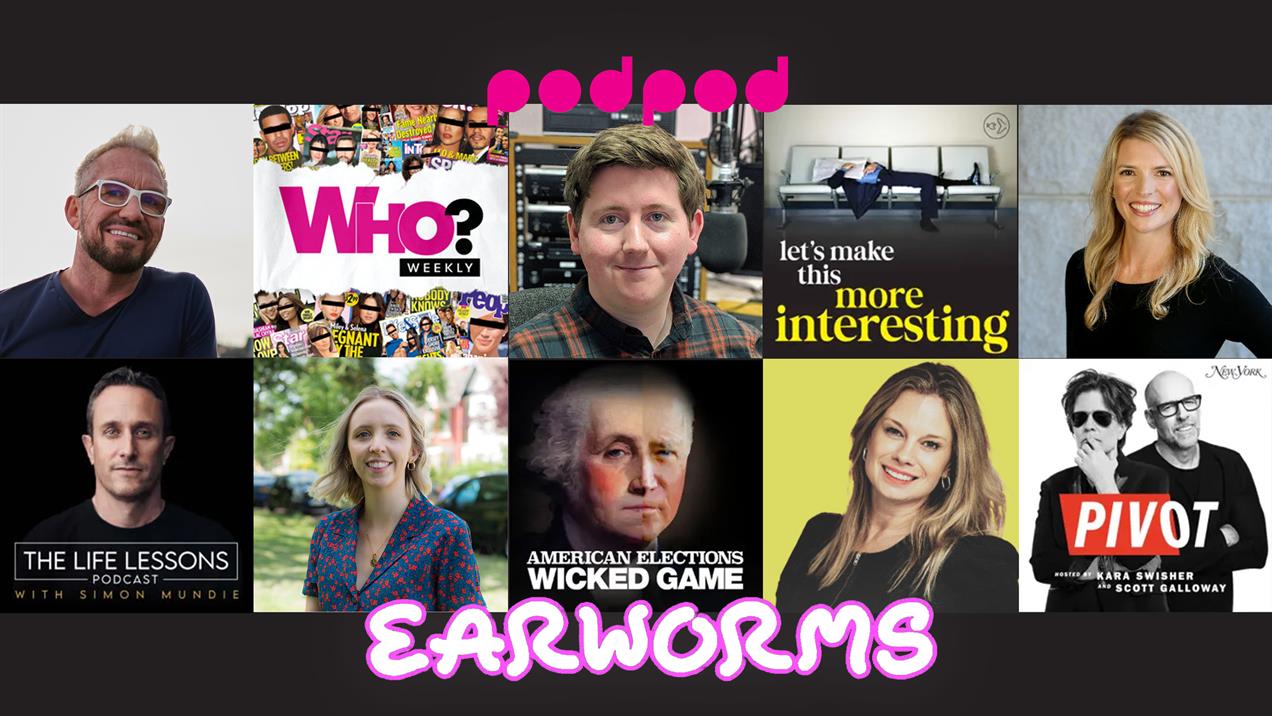The image is a colorful promotional screenshot from a podcast website, featuring a selection of podcasts organized into two rows, each containing five podcasts. The setting indicates an event or a promotional feature showcasing various speakers and their podcasts. The background colors involve a mix of purples, pinks, blacks, reds, yellows, whites, beiges, greens, and blues, bordered by black at the top and bottom.

In the top row, starting from the left:
- The first podcast features a man with white glasses, a blonde mohawk, and a blue shirt.
- Next, there's the “Who? Weekly” podcast.
- The third image shows a man with short brown hair in a plaid shirt, seated in an office.
- The fourth podcast titled “Let’s Make This More Interesting” shows a man lying horizontally on a couch.
- The far right features a blonde woman smiling at the camera, wearing a black long-sleeve shirt.

In the bottom row, starting from the left:
- The first podcast “The Life Lessons Podcast with Simon Mundy” features a man in a black room.
- Next, there is a woman smiling at the camera, dressed in a blue top with red spots, set against a neighborhood backdrop.
- The third podcast, titled “American Election: Wicked Game,” shows an image of a distressed George Washington.
- Fourth from the left is a woman smiling at the camera with shoulder-length brown hair, wearing a black top.
- The last podcast on the bottom right, “Pivot,” hosted by Kara Swisher and Scott Galloway, features two men in black and white, one wearing sunglasses and the other in regular glasses.

The top reads "Pod Pod," possibly in purple-pink text, while the bottom of the image features “Earworms” with a white and pink lettering style.